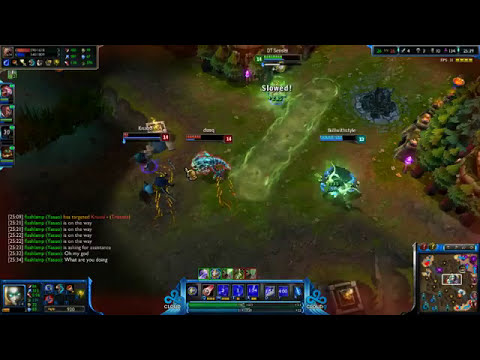This image captures a scene from the isometric, real-time strategy game League of Legends. In the fore-ground, a variety of player-controlled characters are positioned in a bright, grassy field. The image is dense with visual information, including extensive heads-up display elements. Notably, in the bottom right corner, there is a square-shaped mini-map with a brown background and a purple design in the middle. 

The central part of the screen features a panel displaying several action icons, each with a unique artistic design. The bottom left corner showcases a character portrait along with additional player information, such as selectable items. A series of chat messages, displayed in white, pink, and green text, are visible just above this. The top corners of the screen provide further essential game information: the top right corner shows a scoreboard, and the top left corner includes more character portraits.

The gaming scene unfolds in a field segmented by color; the top portion is lush and green, while the bottom part transitions to a darker, brownish terrain. To the right, hedges shape a V, flanked by light structures, adjacent to which are large plasma circles and a plasma cannon. Additionally, red, blue, and green health bars are visible in the middle, indicating ongoing combat amidst the forest-like backdrop.